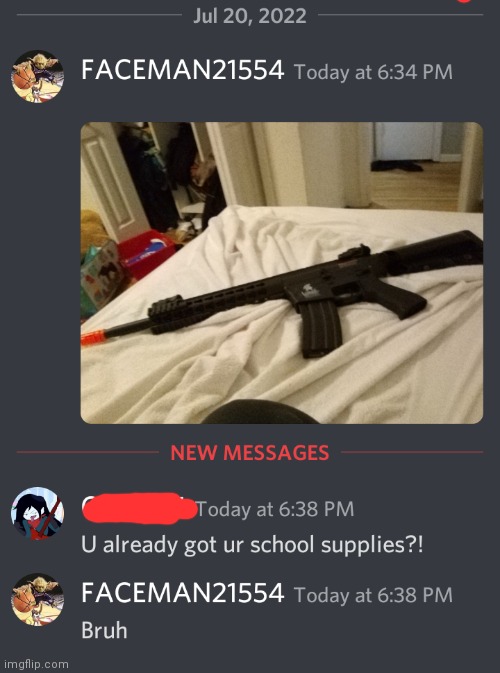The image is a cropped screenshot of the Discord app, most likely taken from a mobile device due to its layout, although this cannot be confirmed definitively as the heads-up display (HUD) is not visible. The identifiable elements in the image, such as the dark gray background and chat interface, confirm it is from Discord. 

The messages within the chat are from two users. The conversation starts with a timestamp indicating July 20, 2022. The first user, named "faceman21554," shares an image of a person holding what appears to be a toy gun. The second user, whose name is obscured, responds with a comment reading, "you already got your school supplies." Subsequently, "faceman21554" replies to this comment with a single word, "bruh."